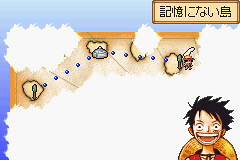The image depicts a screenshot from a video game, heavily stylized with anime-like elements. Prominently positioned in the bottom right corner, a character with spiky black hair and large, expressive eyes is shown grinning widely, revealing rows of white teeth and a visible tongue. The character, dressed in a red tank top and a black necklace, appears animated with spiky bangs partially covering their forehead. A hat is strapped to their back, and they are partially obscured by a white background.

Above them, the screen showcases a map with several brown islands against a dark brown, parchment-like backdrop. These islands are interconnected by blue dots. Notably, on the rightmost island, a small figure stands next to a tree. The upper right corner of the image features a yellow rectangular box with black Asian characters inside, likely Japanese or Chinese text. The rest of the background flows from a lighter blue at the top, progressively darkening towards the bottom left, interspersed with fluffy clouds or a brushed effect.